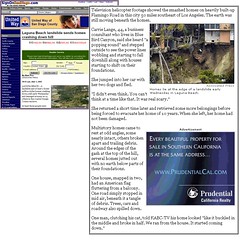This image consists of two screenshots placed side by side, with the one on the left being smaller than the one on the right. The overall image quality is poor, rendering most of the text illegible. The larger portion on the right features a photograph that appears to depict a mudslide or rockslide occurring beneath some residential homes. At the bottom right corner of this section, there is a clearly visible advertisement promoting real estate in Southern California, with the tagline, "Every beautiful property for sale in Southern California is at the same address, www.prudentialcal.com, Prudential California Realty." The remaining portions of both images contain text that is too small and blurry to be deciphered. Notably, there are no animals, birds, bridges, mountains, automobiles, airplanes, helicopters, boats, or trains visible in either of the screenshots.